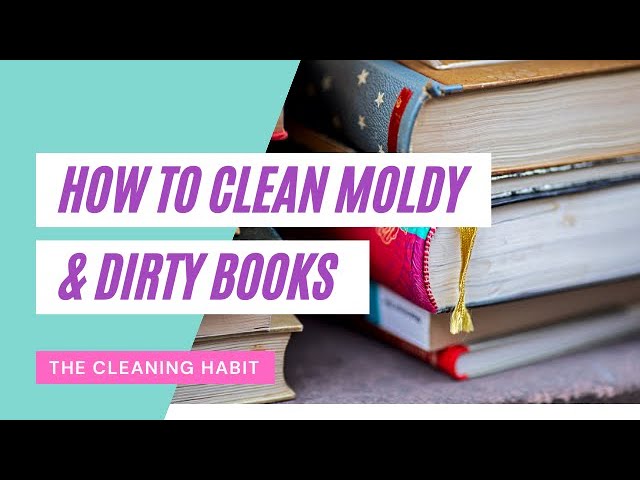This image appears to be a square photograph, enhanced with digital elements. It features a stack of five books positioned on the right side of the frame. The top book is white with a blue spine decorated with white stars. The second book, partially obscured by text, is very thin. Below it is a book with a red spine, followed by a softcover book with a white spine. The bottom book in the stack is another thin volume with a red spine. The left side of the image showcases a light green background with two white rectangular overlays containing text. The top rectangle features purple lettering that reads, "How to Clean Moldy and Dirty Books," while the bottom rectangle holds a pink label that says, "The Cleaning Habit." The photograph is bordered with black bars at both the top and bottom, as well as a narrow white bar just above the bottom black border.